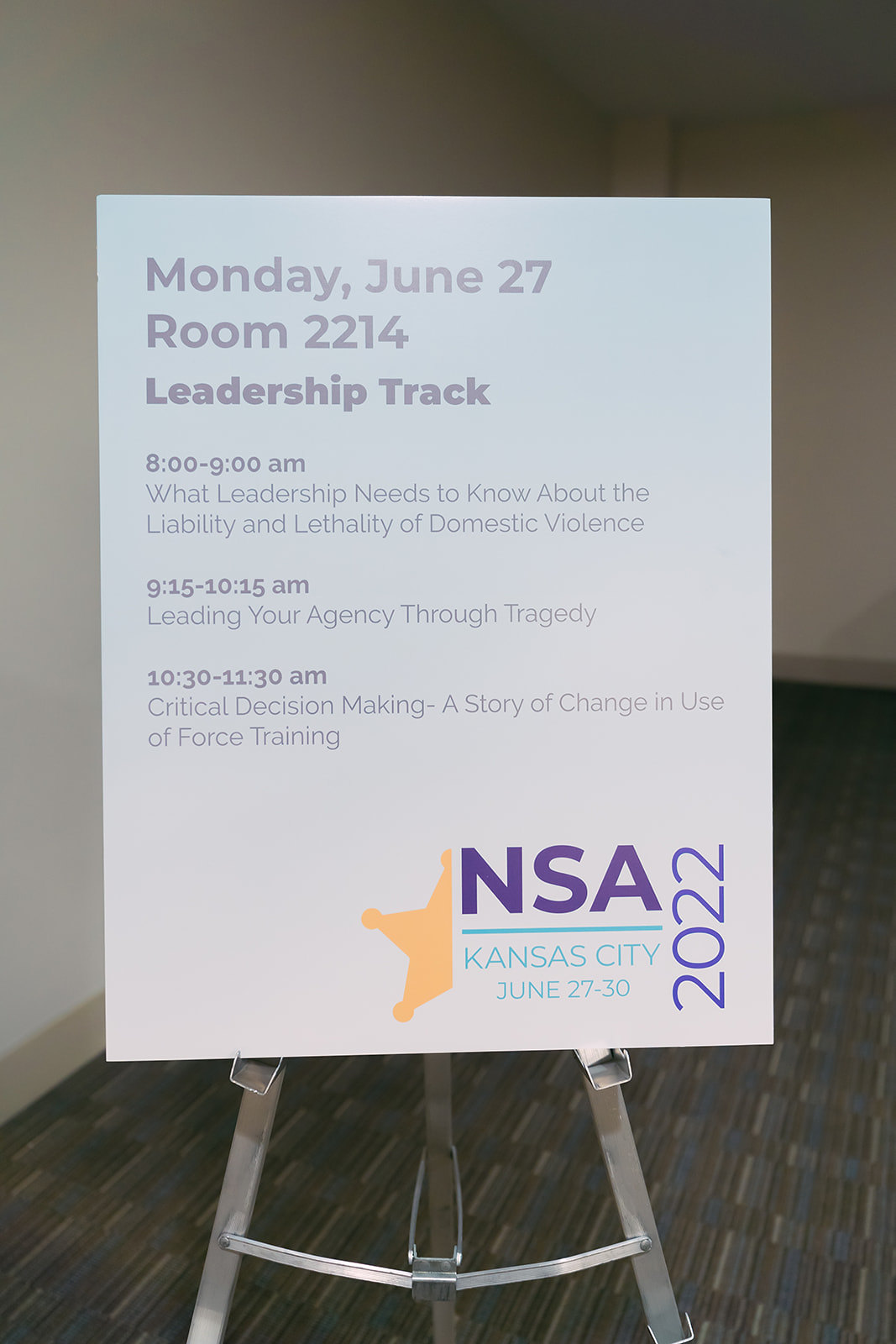The image features a rectangular poster displayed on a silver metallic tripod stand, situated inside a room with white walls and a brown floor accented with various shades of brown and some blue. The poster, set against a light blue background, outlines a schedule for a conference in Room 2214 under the Leadership Track. It reads: "Monday, June 27, Room 2214, Leadership Track, 8:00 to 9:00 a.m.: What Leadership Needs to Know About the Liability and Lethality of Domestic Violence, 9:15 to 10:15 a.m.: Leading Your Agency Through Tragedy, 10:30 to 11:30 a.m.: Critical Decision Making, A Story of Change in Use of Force Training." At the bottom right corner of the poster, there is a logo resembling the left half of a gold star, along with the text "NSA, Kansas City, June 27 to 30, 2022."